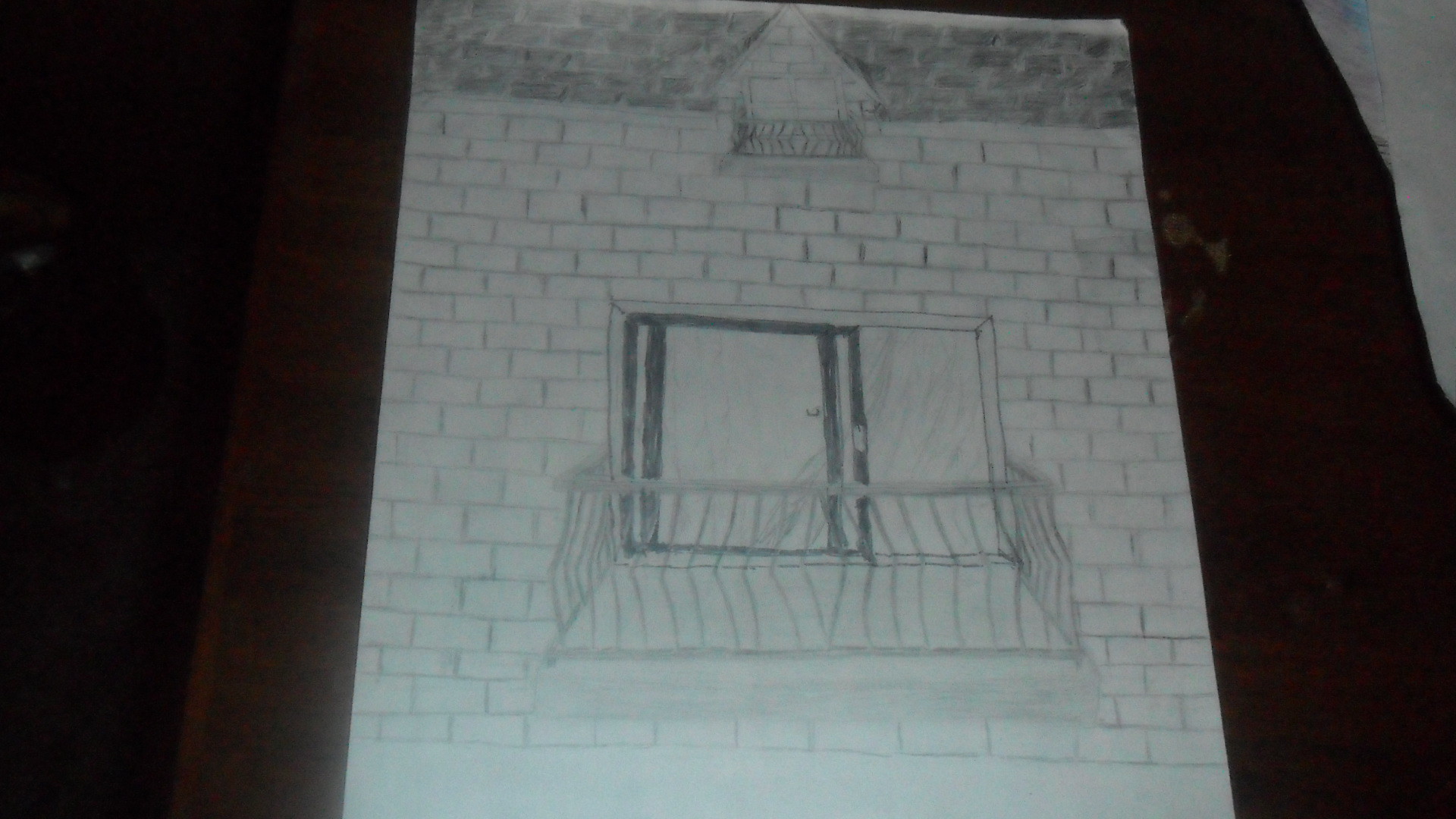This image is a photograph showcasing a pencil sketch on sketch paper, set against a predominantly black fabric background. The sketch intricately depicts the side of a brick house, focusing on architectural details. Central to the drawing is a sliding glass door, partially open to the left, leading to a small balcony surrounded by an uneven iron rail, designed to fit just enough space for a person to stand. Above this, a triangular gable is visible, adorned with what appear to be etched details of flowers or other embellishments. Despite the artistic effort, the proportions of elements like the balcony rails and the door seem inaccurately rendered, with misaligned lines contributing to the impression of a beginner's work or a rough draft. The upper portion of the sketch is lighter, possibly indicating a contrast with the heavier, dark strokes of the lower brickwork, adding depth to the side of the house.